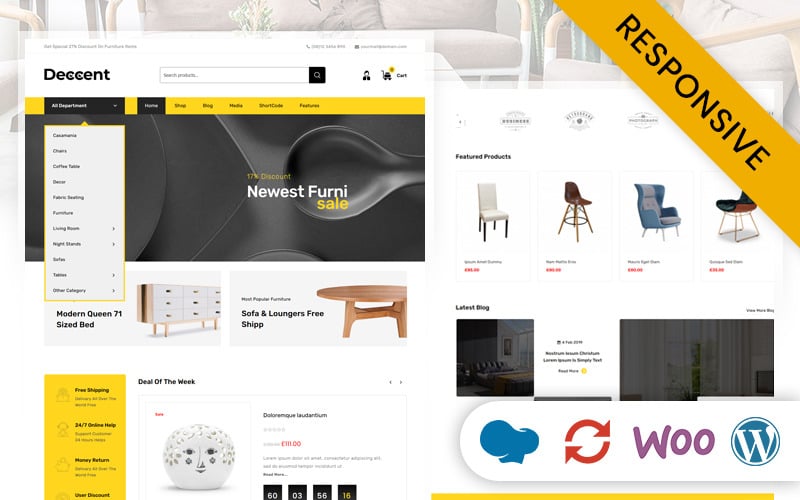Two screenshots from the DECENT (D-E-C-C-E-N-T) website are presented in a collage layout against the backdrop of an elegantly furnished room featuring classy gray-cushioned furniture. The images, slightly dimmed and grayed out, highlight different sections of the site's homepage. 

On the left side of the collage, the DECENT homepage displays various categories, offering a glimpse of modern furniture pieces like a coffee table. However, there are noticeable inconsistencies, with product descriptions not aligning correctly with the items, suggesting the site may still be under development and using placeholder text.

The right side of the collage showcases a selection of contemporary chairs and a decorative ceramic piece, accompanied by text proclaiming "New Furniture Sale" and "Deal of the Week." Additionally, social media links are visible at the bottom right corner, indicating the brand's online presence.